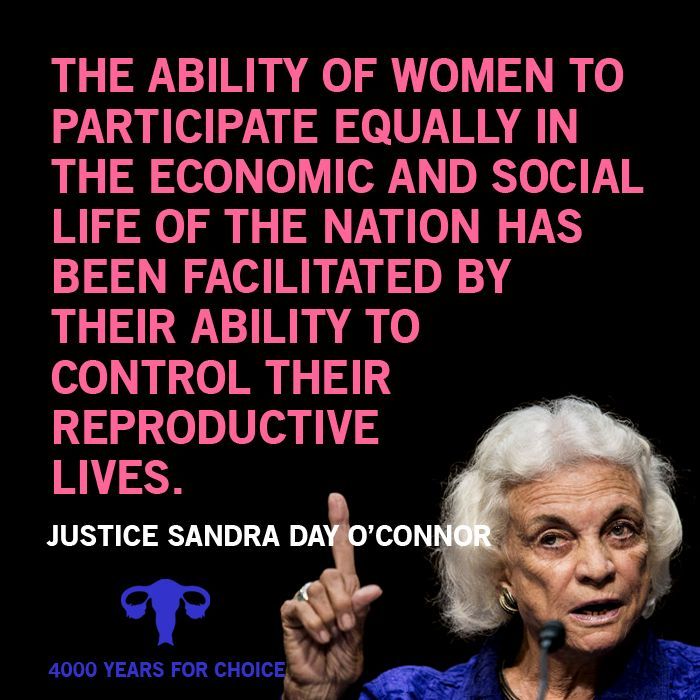The image features a powerful quote by Justice Sandra Day O'Connor, prominently displayed in pink text on a black background. The quote reads, "The ability of women to participate equally in the economic and social life of the nation has been facilitated by their ability to control their reproductive lives." Just below the quote, Justice Sandra Day O'Connor's name is highlighted in white. In the lower right corner of the image, Justice O'Connor is depicted, raising her right hand with her index finger pointed up, speaking into a microphone. She has white hair and is dressed in a blue outfit. To the left of the image, the phrase "4,000 Years for Choice" is displayed, accompanied by a symbol of scales of justice just above it.